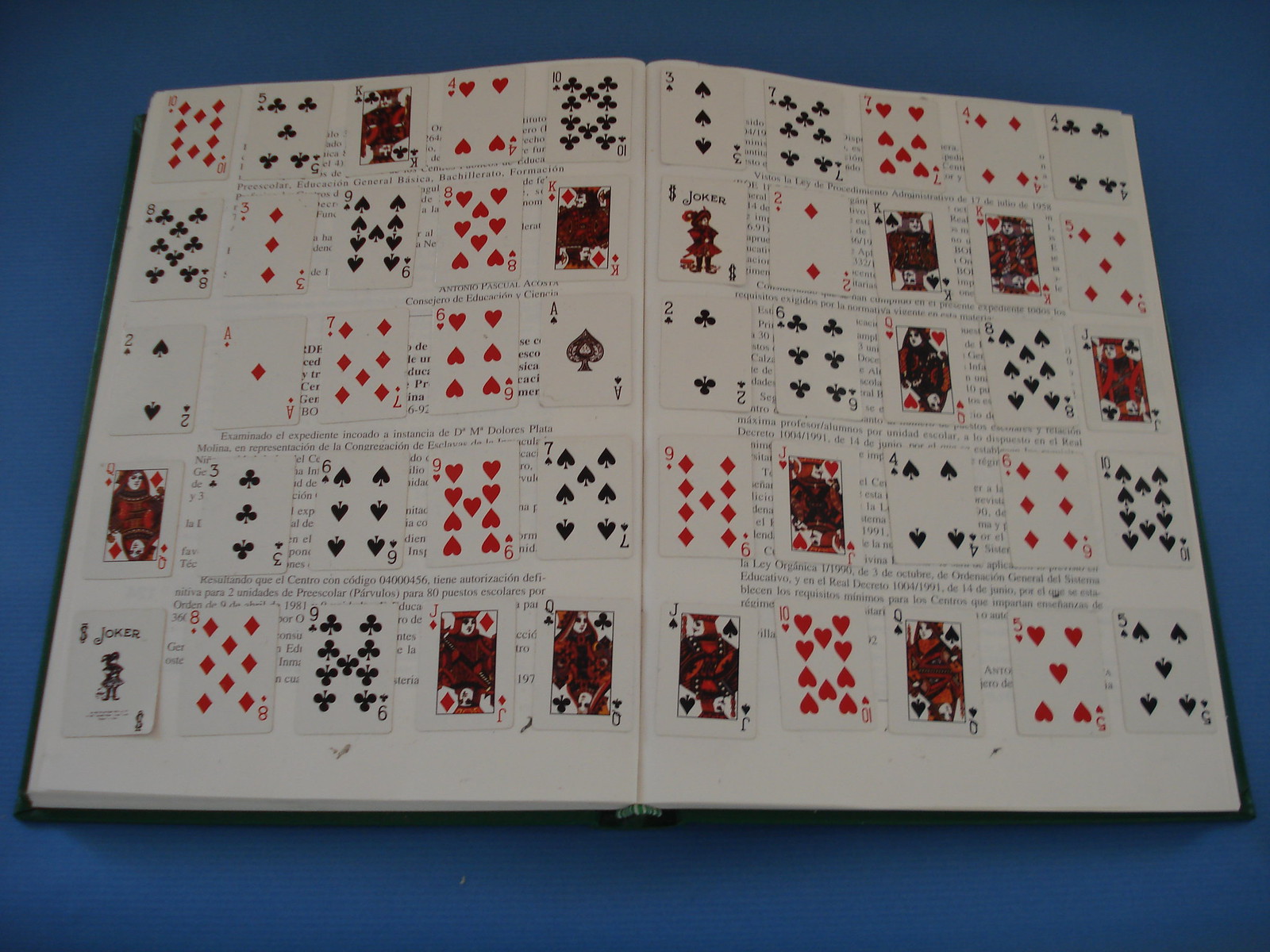The image displays a blue table with a large, black-covered book open to its middle, occupying most of the frame. The book's pages are predominantly white and are covered with an assortment of playing cards arranged in a seemingly random manner. There are five rows and five columns of cards, with each card differing from the next, alternating predominantly between red and black suits. Some visible cards include the 10 of hearts, 5 of clubs, 9 of spades, 4 of hearts, 9 of clubs, 3 of clubs, and 7 of spades. The original text of the book is faintly visible behind the cards, suggesting that they were placed atop the pages without adhering to any apparent logic or pattern. This gives the impression of an impromptu or artistic arrangement. The black cover of the book frames the display, adding to its unique visual appeal.